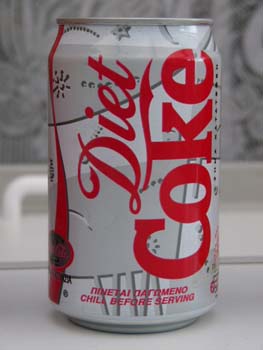This extreme close-up photograph captures a can of Diet Coke set against a white table surface, with a softly blurred background featuring a light gray and white floral-patterned wallpaper. The can stands upright and displays a striking design: a white and gray background adorned with snowflake shapes, spirals, and starbursts, indicative of perhaps an artsy collector's edition. The iconic Diet Coke logo in bold red letters dominates the center of the can. Beneath the logo, small Russian text can be seen, accompanied by the English instruction, "Chill before serving." The dim lighting and tight cropping of the image focus the viewer's attention solely on the intricately detailed can, emphasizing its international origins and unique aesthetic.